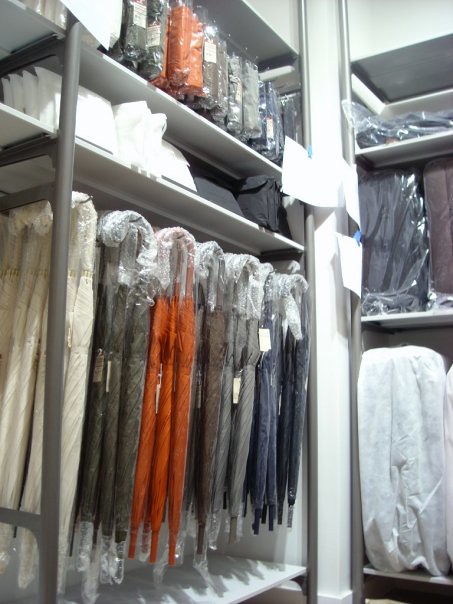The image depicts a modern, brightly lit retail display, likely in a department store. The overall aesthetic is neutral, dominated by white and light gray tones. A variety of items are meticulously organized, some of which are still wrapped in plastic, indicating they are for sale. On the bottom left, several umbrellas hang on hooks, in a color gradient that includes cream, dark brown, pumpkin orange, lighter brown, light gray with a blue tint, regular blue, and navy blue. Above the umbrellas, folded items in rectangular shapes sit on a shelf, with more packaged goods in the same color scheme on higher shelves. To the right, three shelves hold plastic-wrapped packages of varying sizes. The largest package at the bottom appears to be wrapped in cotton, with additional plastic-wrapped pieces above it, possibly luggage or similar items. The standout color among the predominantly monochromatic scheme is orange, offering a vibrant contrast to the overall decor.